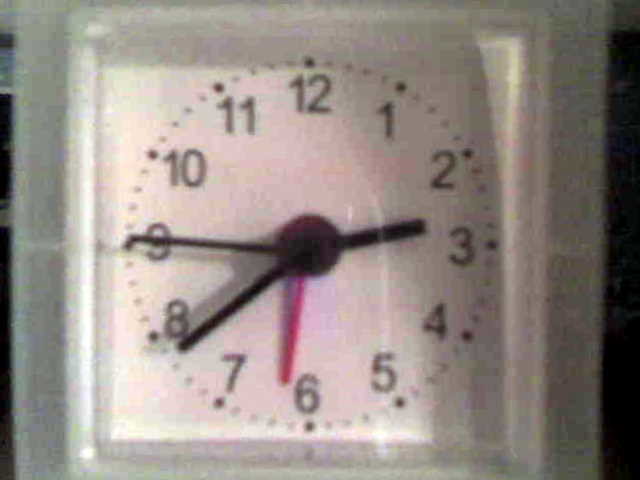This zoomed-in image features a clock with a unique design. The clock itself is circular, set within a square frame. The outer edges of the image are predominantly black, heavier on the right side and narrower on the left. A gray border frames the clock within the square.

The clock face inside shows a detailed layout with black dotted lines marking each numeral, accompanied by the respective numbers: 12 at the top, followed by 1, 2, and 3 on the right, 4, 5, and 6 at the bottom, 7, 8 leading up to 9 on the left, and 10, 11 back up to 12. Between each numeral, there are four dashed lines indicating the 15-minute increments.

The clock hands are distinctively colored: both the shorthand (hour) and longhand (minute) are black, while the seconds hand is red. In this particular moment, the minute hand points directly at the 9, the hour hand is positioned between the 7 and 8, and the seconds hand is just past the 6.